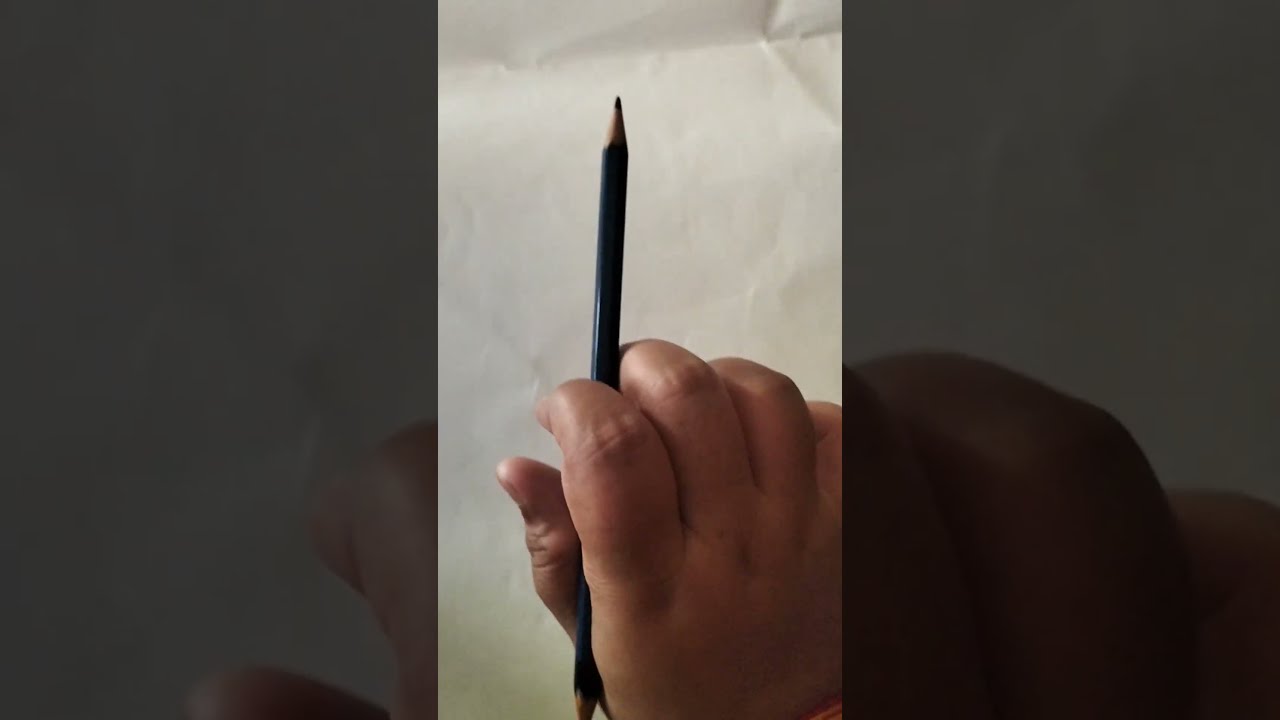The image is a vertical, cell phone-style screen grab of a video featuring a brown-skinned hand holding a double-sided, dark-colored drawing pencil. The hand, which appears childlike and is characterized by thick fingers and baby fat, positions the pencil between the meaty part of the thumb and the pointer and middle fingers, roughly halfway down its length. The pencil is sharpened on both ends. The background of the image is largely occupied by a blank, white, wrinkled sheet of paper with crinkles more prominent around the corners and faint shadows, particularly in the upper edge. This scene is framed within a second blurred and faded close-up of the hand's knuckles in grayscale, giving the impression of a layered or zoomed-in background. The elevated, slightly angled camera perspective suggests the hand is poised, possibly indicating the beginning of a drawing session or an instructional video setup, akin to something you might find on a platform like TikTok.